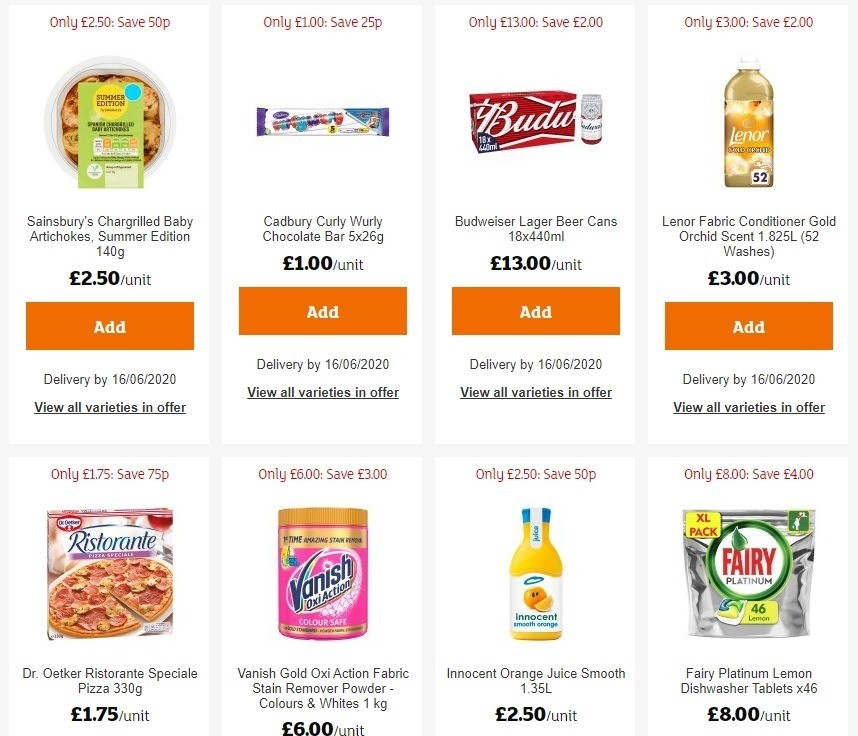This image is a detailed screenshot from an unidentified e-commerce grocery shopping website, which features a white and orange color scheme. The website has a clean, white background with prominent orange buttons labeled "Add" in white text for adding items to the shopping cart. The layout displays products in a grid format, with two rows and four items per row.

In the top row, the first item is "Sonsberry Char-Grill Baby Artichoke Summer Edition," available in 140 grams and priced at 2.5 pounds per unit, shown in a plastic case resembling cookies. Next to it is "Cadbury Curly Whirly Chocolate Bars," which appears as a typical candy bar in its image. The third item is "Budweiser Lager Beer Cans," sold in red cardboard cases, priced at 13 pounds per unit. The final item in the top row is "Lenora Fabric Conditioner Gold Orchid Scent," priced at 3 pounds per unit.

Accompanying each product is a clear image depicting the respective item, contributing to a visually navigable online shopping experience.